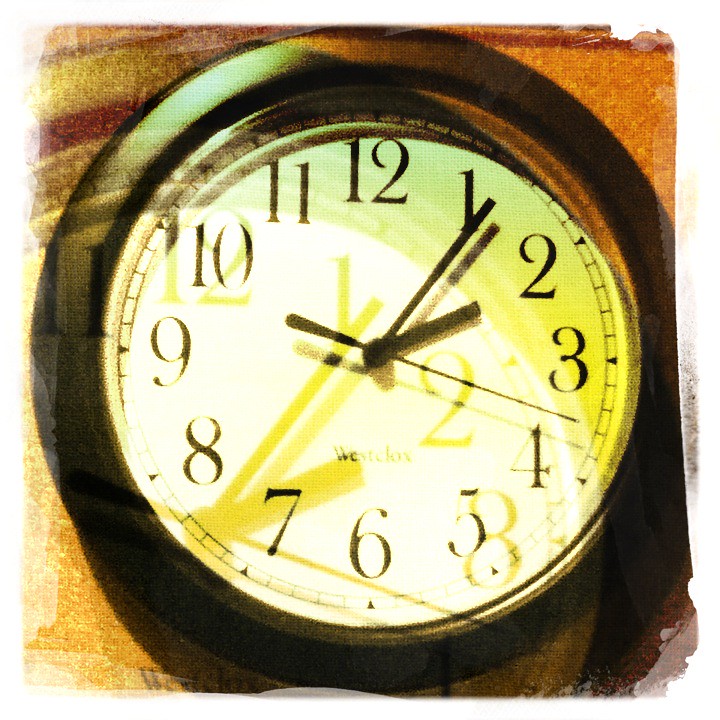The image depicts a round analog clock with a black frame and white dial, prominently showing the time as 2:06:18. The clock features black hands and clearly labeled numerals from 1 to 12. Surrounding the dial is a circlet of small rectangles between the numbers and the clock's border. The depth and shadowing effects on the clock's frame suggest careful lighting, accentuating its design. Superimposed over the primary clock is an enlarged, semi-transparent shadow image of another clock, or possibly the same one, aligned perfectly to match the original clock's time and hands. This gives a layered visual effect, revealing evident digital editing around the image's borders. The background appears to be a wood texture, although it seems digitally altered, potentially painted, adding to the image's artistic and edited ambiance.